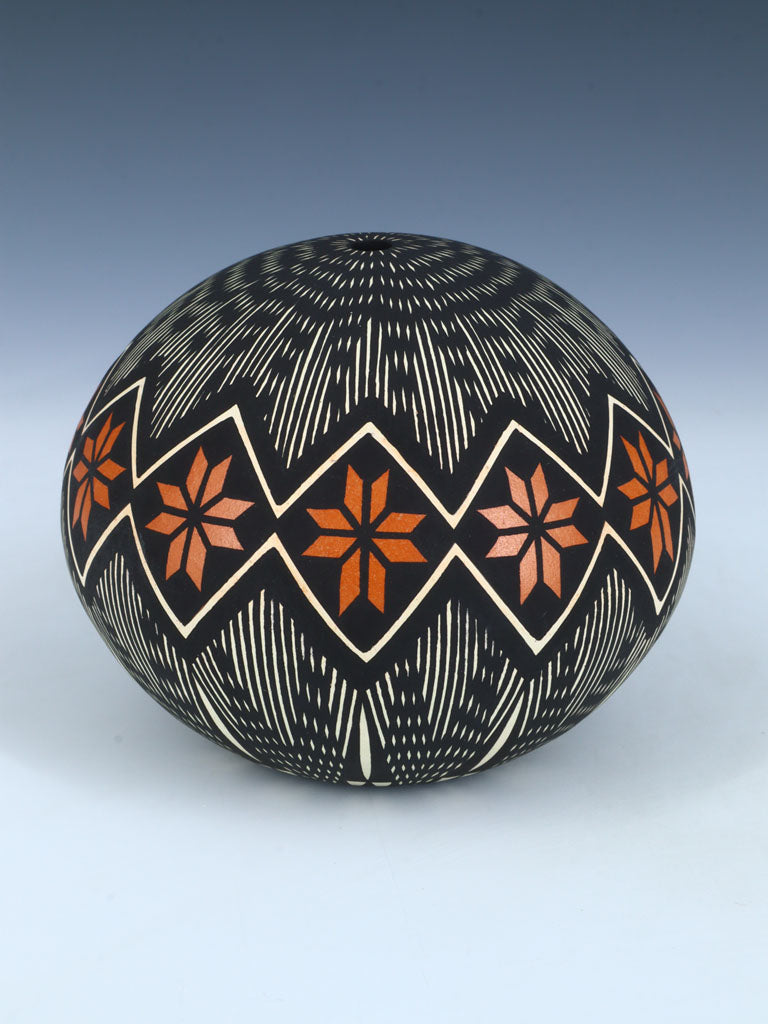The image showcases a decorative spherical object, reminiscent of a piece of art or pottery, placed on a pastel blue table with a bluish-white background. The sphere, slightly squished at the poles, features a complex design of black and white lines interwoven like hairs, forming a textured weave. Prominently displayed are five red or orange flower-like crosses, evenly spaced around the sphere, each seated within a black diamond pattern that accentuates their vivid color. These crosses have intersecting lines within, giving the appearance of a stick figure at each vertex. Encircling the crosses are zigzagging thin white lines and thicker black lines mimicking a frequency waveform, adding dynamism to the design. The art piece appears to reflect early Native American pottery styles, emphasizing its cultural richness and geometric precision.